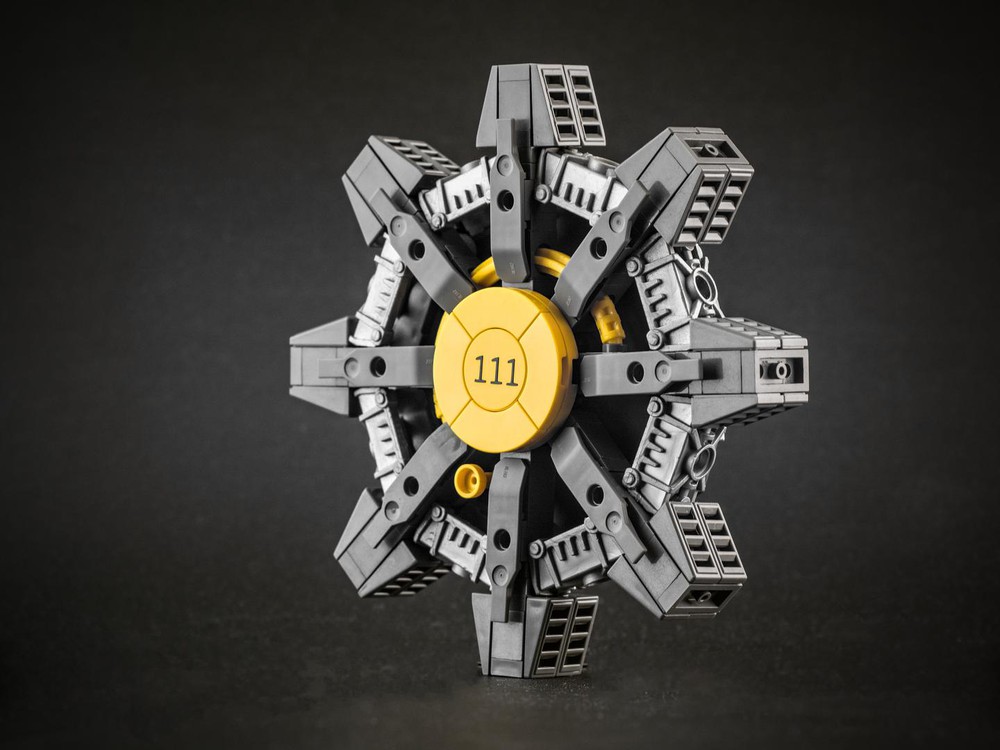This image displays a digitally generated design of a gear wheel. The main gear wheel is depicted vertically and is predominantly gray in color. Around the circumference of the gear, there are eight evenly spaced, three-dimensional trapezoidal projections, all in shades of gray. Each trapezoid features a section with eight small, square cutouts, contributing to the intricate design.

In the foreground, the wheel shape is highlighted, appearing circular with seven or eight gray, belt-like straps encircling it. These straps resemble plastic and each has a black hole at its center. At the very core of the gear, a circular emblem bears the number "111". Behind this numeral is a curved yellow line, adding a burst of color to the design, while a yellow plug appears prominently in front of the emblem.

The background of the image is a gradient mix of black and gray hues, which contrasts with and accentuates the details of the gear wheel. The overall composition creates a visually striking representation of a mechanical component, blending both functional design and artistic elements.